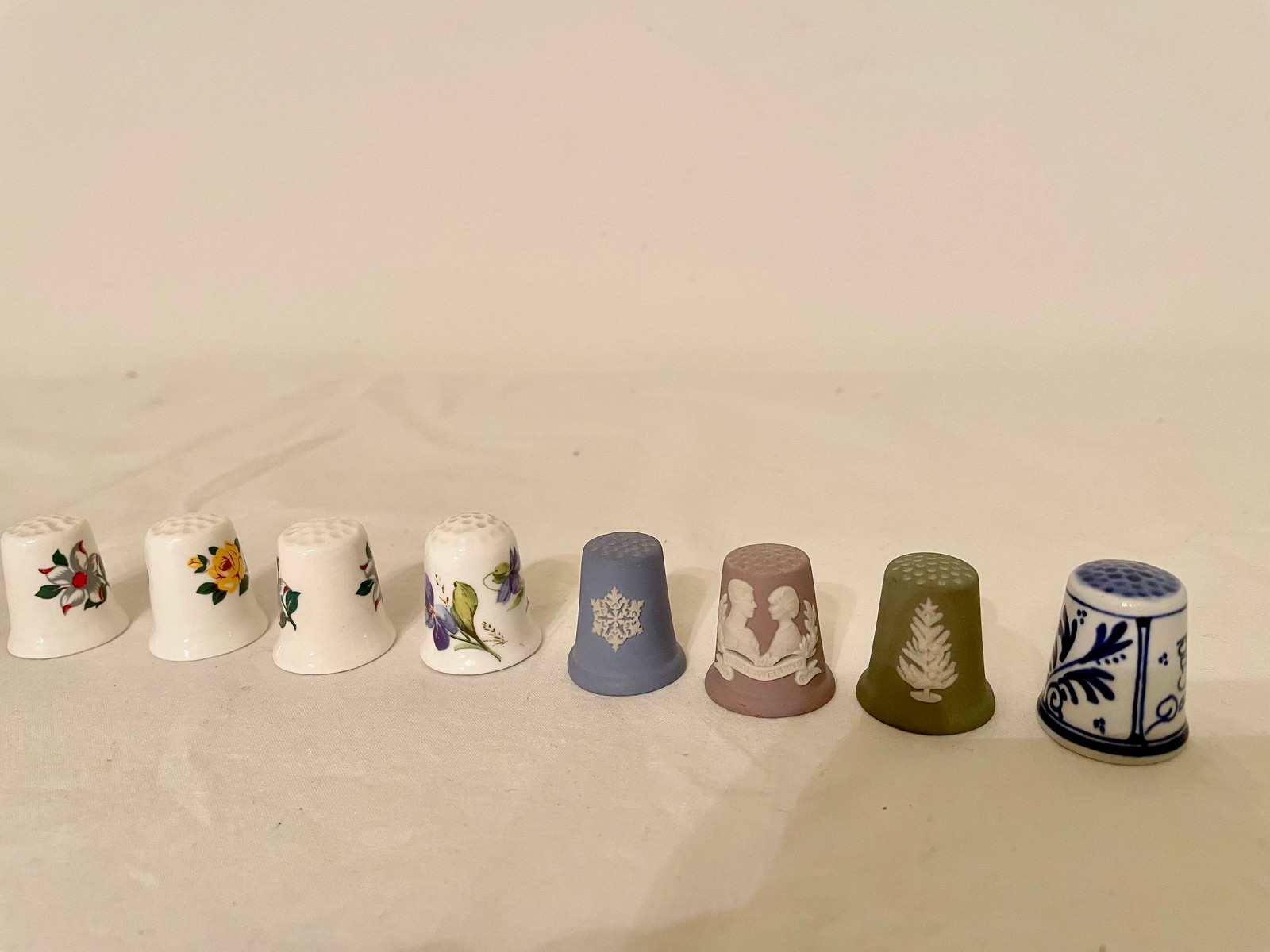This photograph showcases a charming collection of eight ceramic sewing thimbles, each beautifully adorned with unique colors and patterns. Arranged on a pristine white cloth, the thimbles present a delightful array of designs. Starting from the left, the first thimble features a white flower with red edges, a red center, and green leaves. Next to it is a thimble with a vibrant yellow rose accompanied by green leaves. The third in line is an off-white thimble displaying leaves on both sides. The fourth thimble, also white, is decorated with delicate green leaves and purple flowers. 

Moving towards the right, we encounter a light gray-blue thimble showcasing a white snowflake in its center. Beside it is a mauve thimble highlighting the silhouettes of a man and a woman facing each other, framed with an emblem and ribbon below. Next comes an olive-green thimble adorned with a white Christmas tree. The final piece in this charming collection is a blue and white thimble featuring intricate floral motifs, dots, and lines. Together, these thimbles create a visually pleasing and diverse display of craftsmanship.